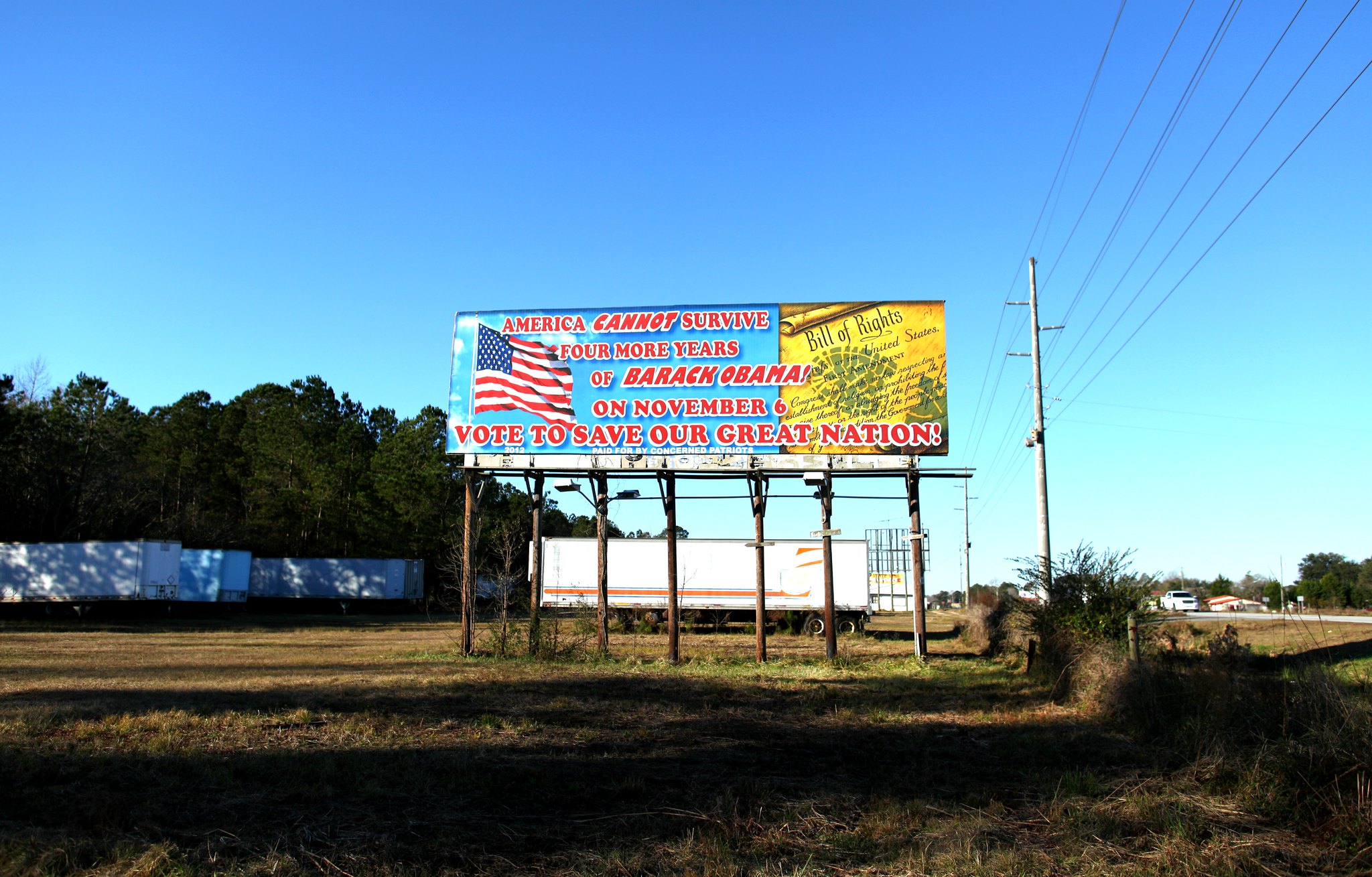In this photograph, there's a weathered billboard standing prominently in the middle of a grassy field, surrounded by unused trailers that connect to semis, all parked behind it. The billboard, supported by wooden poles, is set against a beautiful, clear blue sky on a bright, sunny day. It features a blue and yellow background with an American flag fluttering on the left side and a fragment of the Bill of Rights, written on yellow paper, on the right. The bold red text on the billboard reads, "America cannot survive four more years of Barack Obama. On November 6th, vote to save our great nation." In the background, a lush green forest is visible, with telephone poles and electrical wires running parallel to a road on the right-hand side of the image. The scene feels distinctly rural, adding to the impression that this political message might be targeting a local, likely conservative, audience.